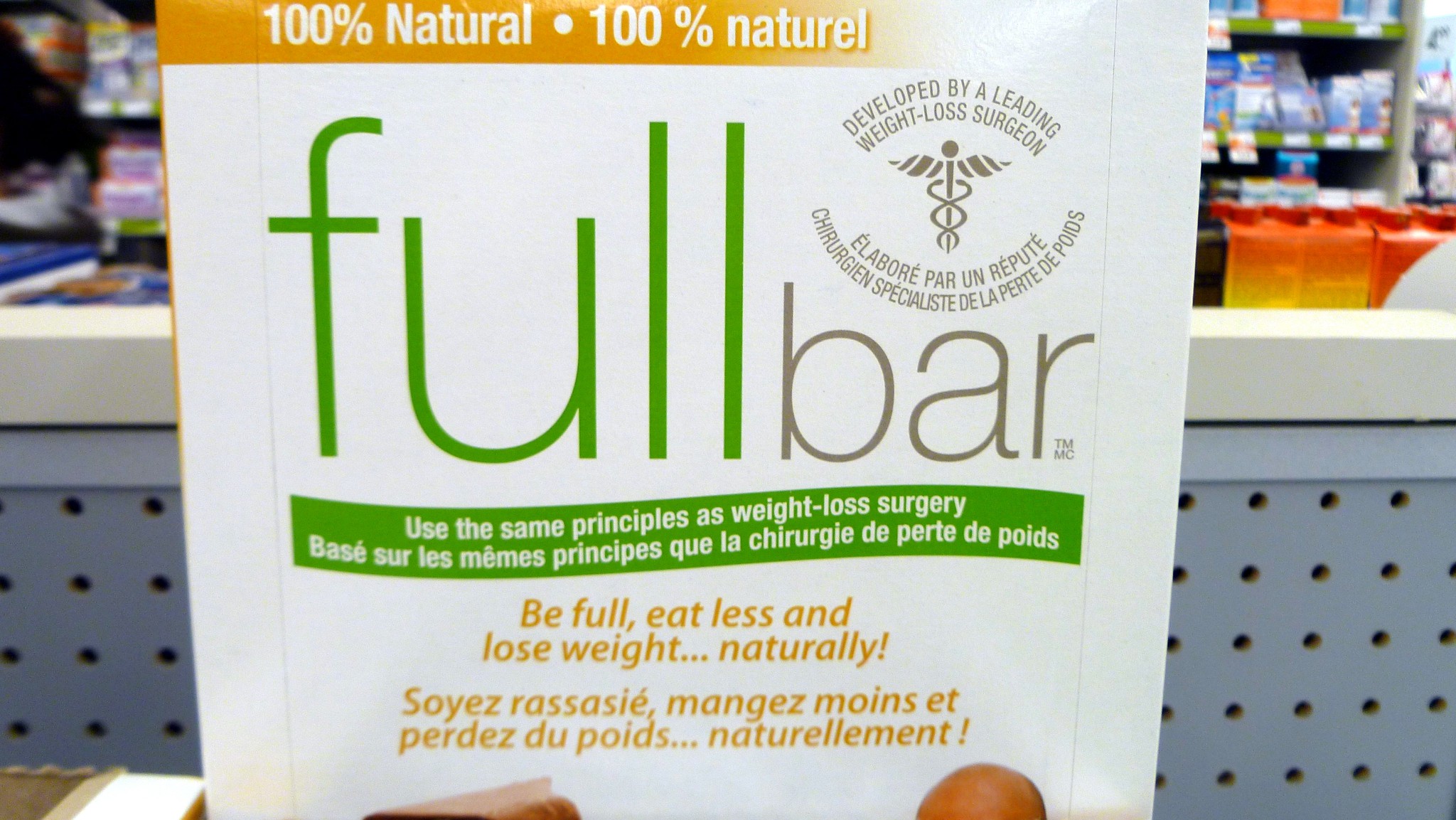A close-up photograph captures a package of Fulbar, a nutritional supplement designed to aid in weight loss by employing principles similar to those used in weight loss surgery. The packaging is prominently displayed, featuring text in English, Spanish, and French that emphasizes its benefits: "Be full, eat less, and lose weight naturally." The package also highlights that the product was developed by a leading weight loss surgeon, indicated by a specific surgeon's symbol. The package primarily showcases a white background with accents of green and gray, and some banners in a butternut squash color.

The Fulbar package is partially cut off at the bottom, suggesting it is positioned on a typical pharmacy shelf, distinguished by its perforated design—a common sight at stores like Walgreens. In the background, additional shelves are visible, lined with blue medical packages accented in white and red, indicating a well-stocked pharmacy setting. This photograph appears to have a glossy finish, emphasizing the clinical and professional environment in which Fulbar is sold.